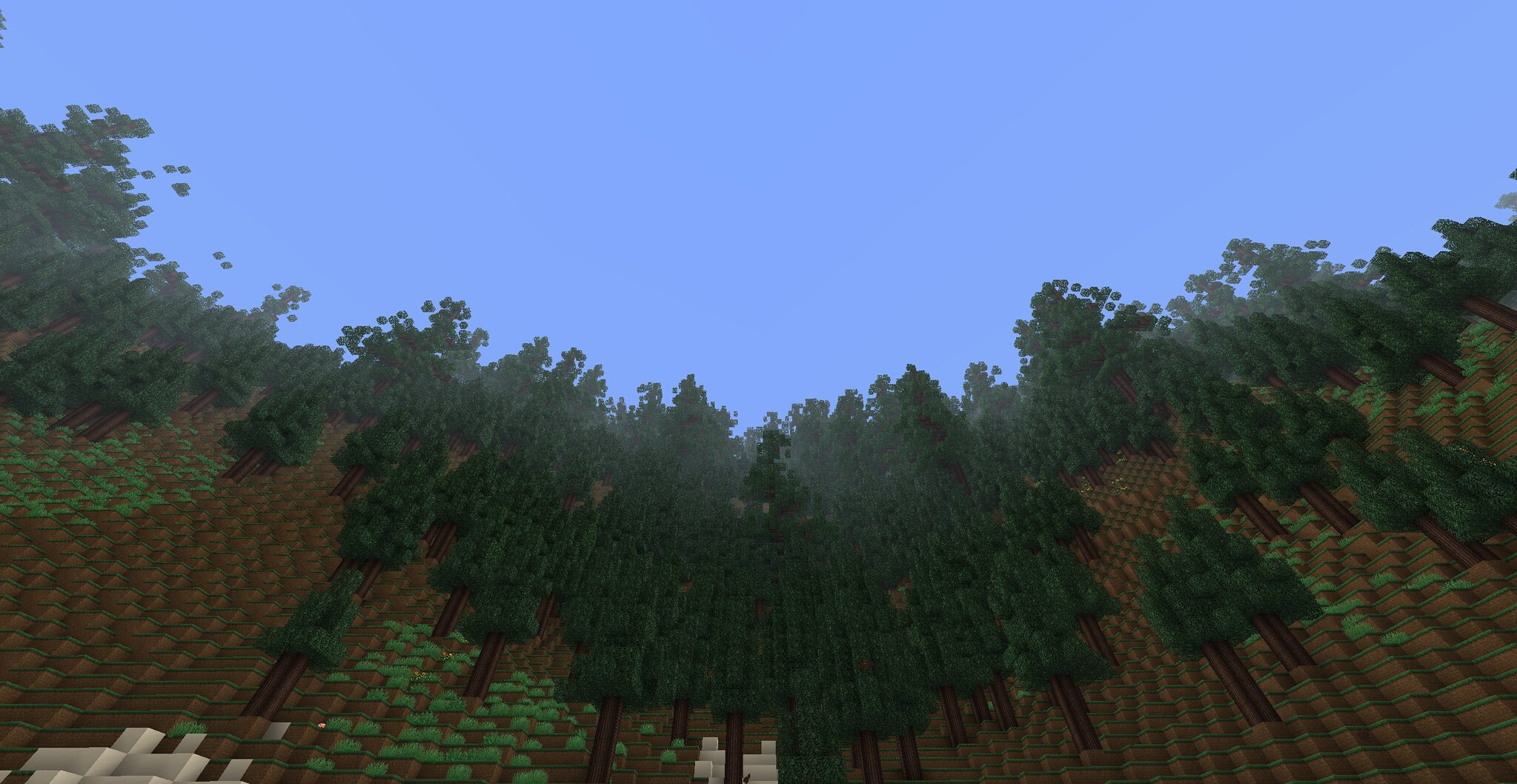This image, likely a screenshot from the game Minecraft, displays a detailed, pixelated outdoor scene. Dominating the background is a bright blue sky. A forest climbs up the side of a mountain, creating a sense of height and vastness. The landscape features raised, textured ground composed of repeating brown blocks topped with green grass, forming an upward diagonal slope. Scattered throughout are taller patches of grass on various sides of the blocks. Within the scene, dark green trees, standing four to five blocks tall, further enhance the verticality and depth of the forest. Brown tree trunks are clearly visible, and their canopies, formed by small rectangular and square leaves, extend into the sky. Additional details include patches of sparse green vegetation, some grey areas resembling large rocks at the lower left, and bright green shapes near the bottom, contributing to the richness of the environment.